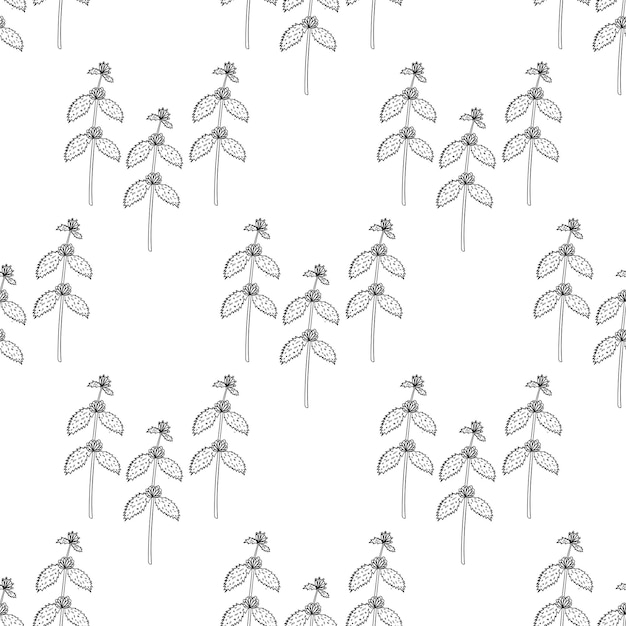The image depicts a meticulously hand-drawn, black-and-white wallpaper or textile pattern, characterized by its simplistic yet appealing design. The pattern consists of an arrangement of thin stems, each adorned with thorny leaves and topped with delicate, tiny blooms. These stems are organized in repeating groups of three. This triplicate motif is repeated evenly across the entire image, forming a diamond pattern that leaves negative space in the center of each diamond, creating a balanced and deliberate design. Upon closer inspection, the pattern exhibits a structured layout spanning five rows: the top row has three plants, the second has two, the third again has three, the fourth has two, and the fifth has three. Each plant shows a careful arrangement of thorns and detailed dots on the leaves, further emphasizing its intricate simplicity. The design is universally versatile, potentially suitable for wallpaper, blankets, sheets, or upholstery.